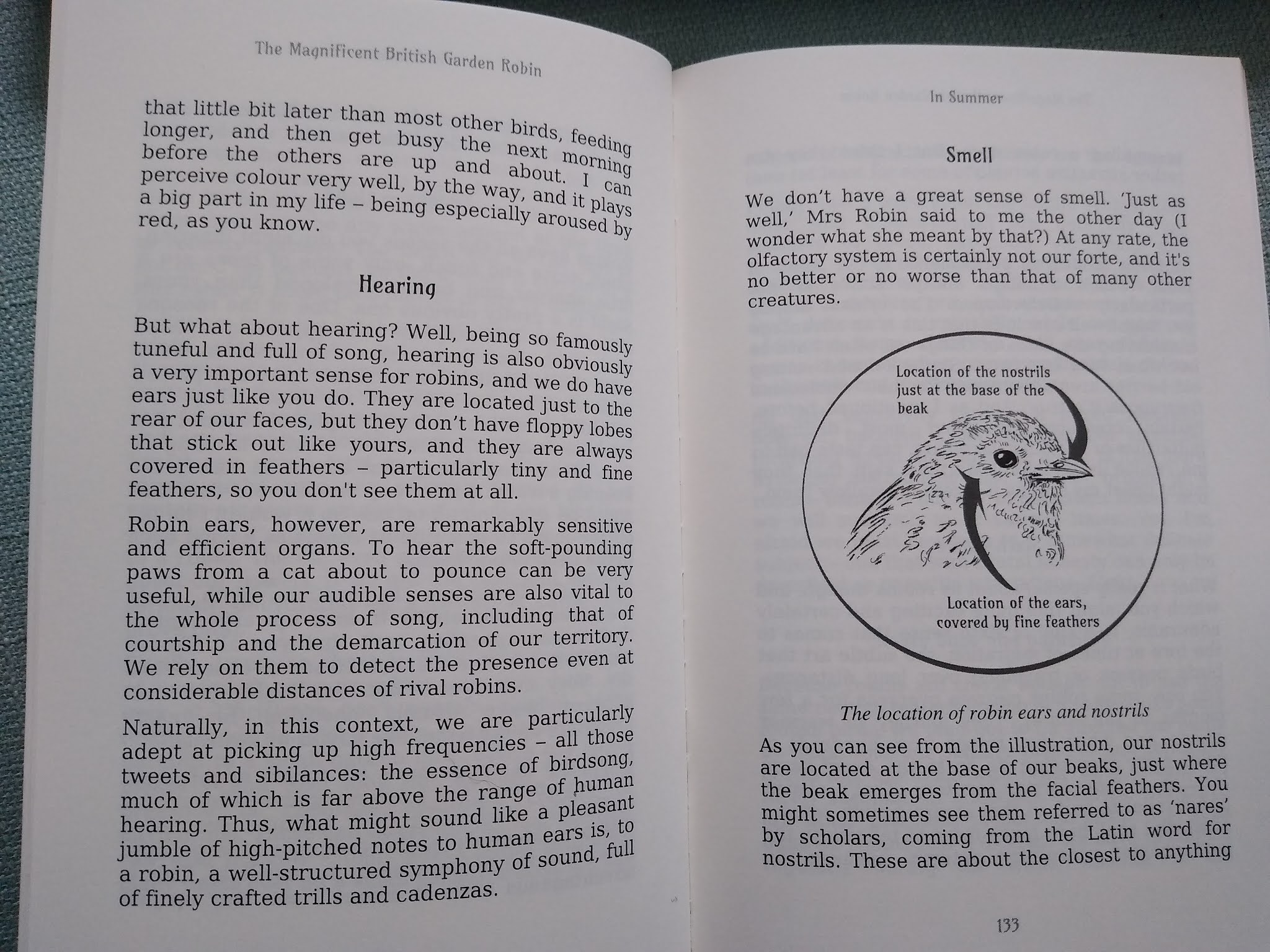The image displays an open book titled "The Magnificent British Garden Robin," with the pages spread on a dark blue fabric. The book is open to pages 132 and 133. The left page is headed by "The Magnificent British Garden Robin" and the word "Hearing," detailing the auditory capabilities of the robin through three paragraphs of text. The right page is headed by "In Summer" and "Smell," containing two paragraphs that describe the robin's olfactory senses. In the middle of the right-hand page, there's a black-and-white circular illustration of a robin's head. The illustration is annotated with "Location of the Nostrils Just at the Base of the Beak" and an arrow pointing to the base of the beak. Another annotation reads "Location of the Ears Covered by Fine Feathers," with an arrow pointing to an area beneath the eye. The overall layout of the pages is clean, with black text and a simple ink drawing, providing a detailed yet straightforward depiction of the robin's sensory anatomy.